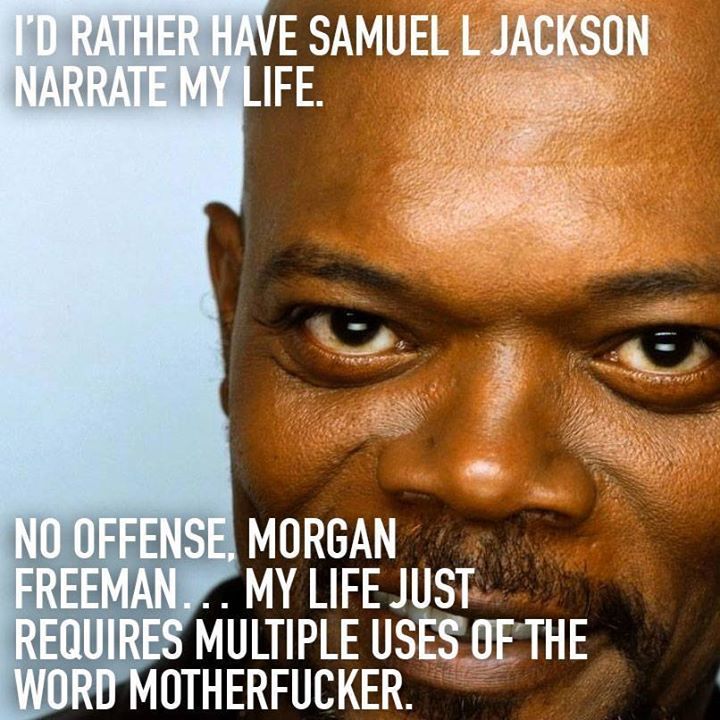This image is a very close-up shot of Samuel L. Jackson's face, where the top of his head, left ear, and part of his chin are cropped out. He is slightly off-center against a light blue background. Jackson's expression is mildly intense, almost a smirk, giving him an air of intensity. He has dark skin, a short black goatee, and a mustache. At the top of the image, in white font, it reads, "I'd rather have Samuel L. Jackson narrate my life." At the bottom, it humorously adds, "No offense, Morgan Freeman, my life just requires multiple uses of the word motherfucker."